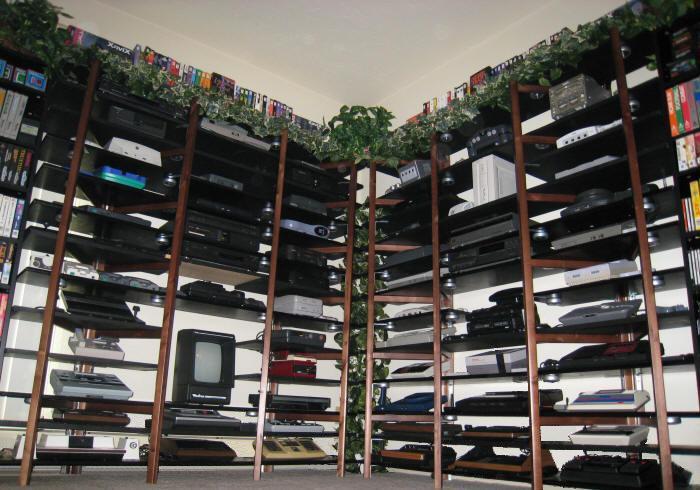The color photograph depicts two large shelving units arranged at a wide angle in front of white walls, creating a makeshift library-like setting for vintage technology. Each shelving unit features approximately 12 to 14 rows stacked vertically, housing a vast collection of old video game consoles and possibly some computer equipment. The devices appear to span from the late 1960s through the 1980s, showcasing various iterations and versions of gaming history. At the top of these shelves, a line of green plants adds a touch of nature, while numerous boxes, likely containing video games or accessories, are neatly placed alongside. This image captures a nostalgic ensemble of technological evolution over decades.